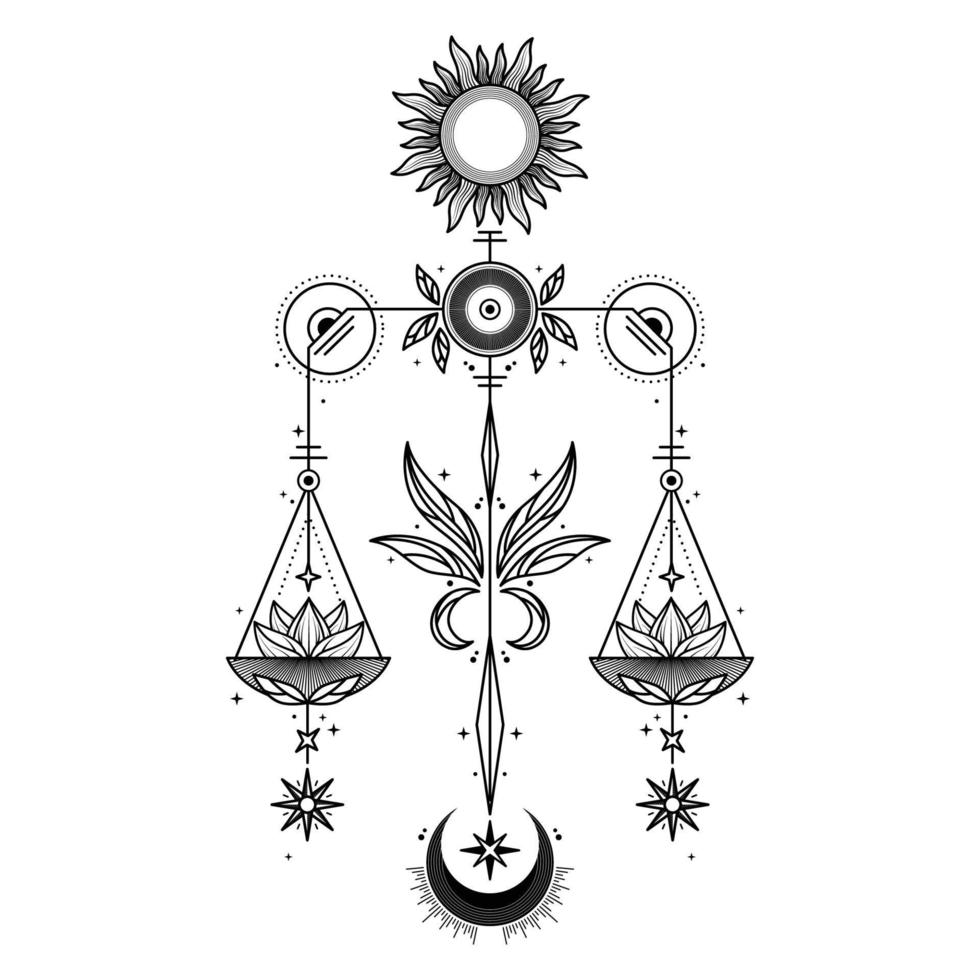This image is a highly detailed black and white line art illustration of a decorative scales of justice symbol, set against a plain white background. The composition, which is roughly four to five inches high and three inches wide, is in portrait orientation. At the very top, a sun-like emblem features a white center encircled by a gray band and a thin black outer line, with wavy gray rays emanating from it.

Directly beneath the sun, two small horizontal lines extend from a central vertical line ending at a prominent circle. This circle is outlined in alternating black and white rings and adorned with three leaf-like shapes on either side. Extending outward from this central circle are two thin black lines leading to two smaller circles on the left and right. These connections curve downwards into the scales themselves.

Each scale descends from a vertical line and features a triangular outline, containing intricate lotus flower designs. Hanging beneath each lotus flower are small star shapes, resembling dangling earrings or delicate ornaments. The scales are visually balanced with identical structures on both sides.

In the centralized lower segment of the image, between the scales, lies an elaborate fleur-de-lis-like symbol. Directly beneath this flourish is a pendant with a crescent moon and a star in its center, adding to the celestial theme.

Overall, the illustration embodies a harmonious blend of geometric and organic elements, depicting a balanced and intricate scales of justice motif.